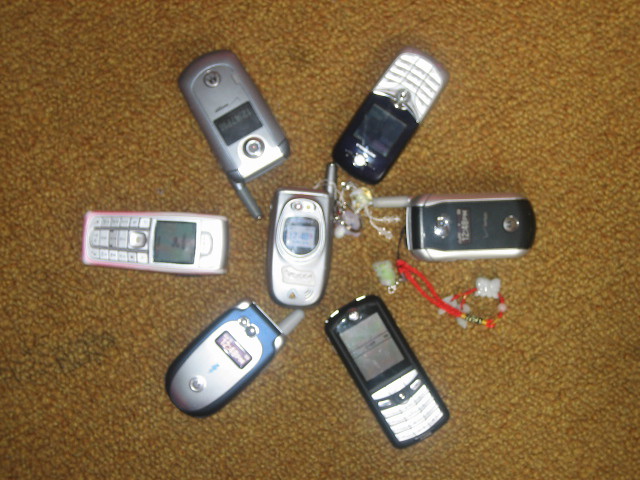In this photograph, a collection of seven vintage cell phones is artfully arranged on a brown Berber-like carpet. The centerpiece of this display is a silver flip phone, with six other phones fanning out around it in a circular, flower-like pattern. Each of these surrounding phones is angled so that their tops, or antennas when present, point toward the central flip phone. The phones are mostly black and silver, but the assortment includes a few with unique touches of color—one with hints of pink on the far left, and another with accents of blue and silver, as well as one with a red string and decoration attached. Though the image is somewhat blurry and the branding on the phones is indiscernible, the overall display showcases the diversity of older mobile phone designs.